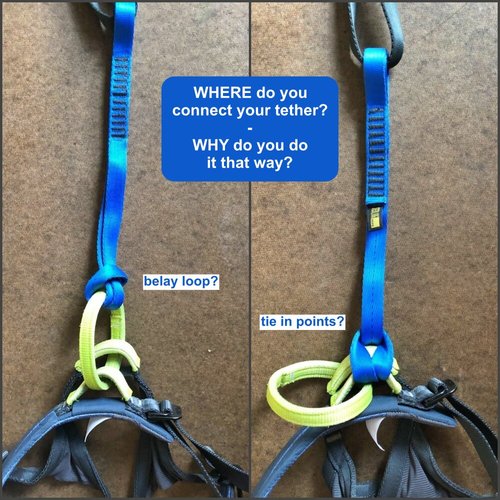The image displays a comparative diagram of two ways to connect a tether, set against a brown background. On the left side, the diagram features a tether colored in blue, green, and black, looping through what is labeled as the "belay loop" in blue text with a question mark. This side shows the tether's black and green sections threaded through each other. On the right side, the image mirrors the same tether, also in blue, green, and black, connecting to what is specified as the "tie-in points," again with a blue question mark. Here, the green loop is positioned horizontally and does not pass through the blue section of the tether. Central to both images is a blue box with white text posing the questions: "Where do you connect your tether? Why do you do it that way?" The images emphasize the distinctions in tethering via belay loop versus tie-in points, illustrating key differences in their configurations.